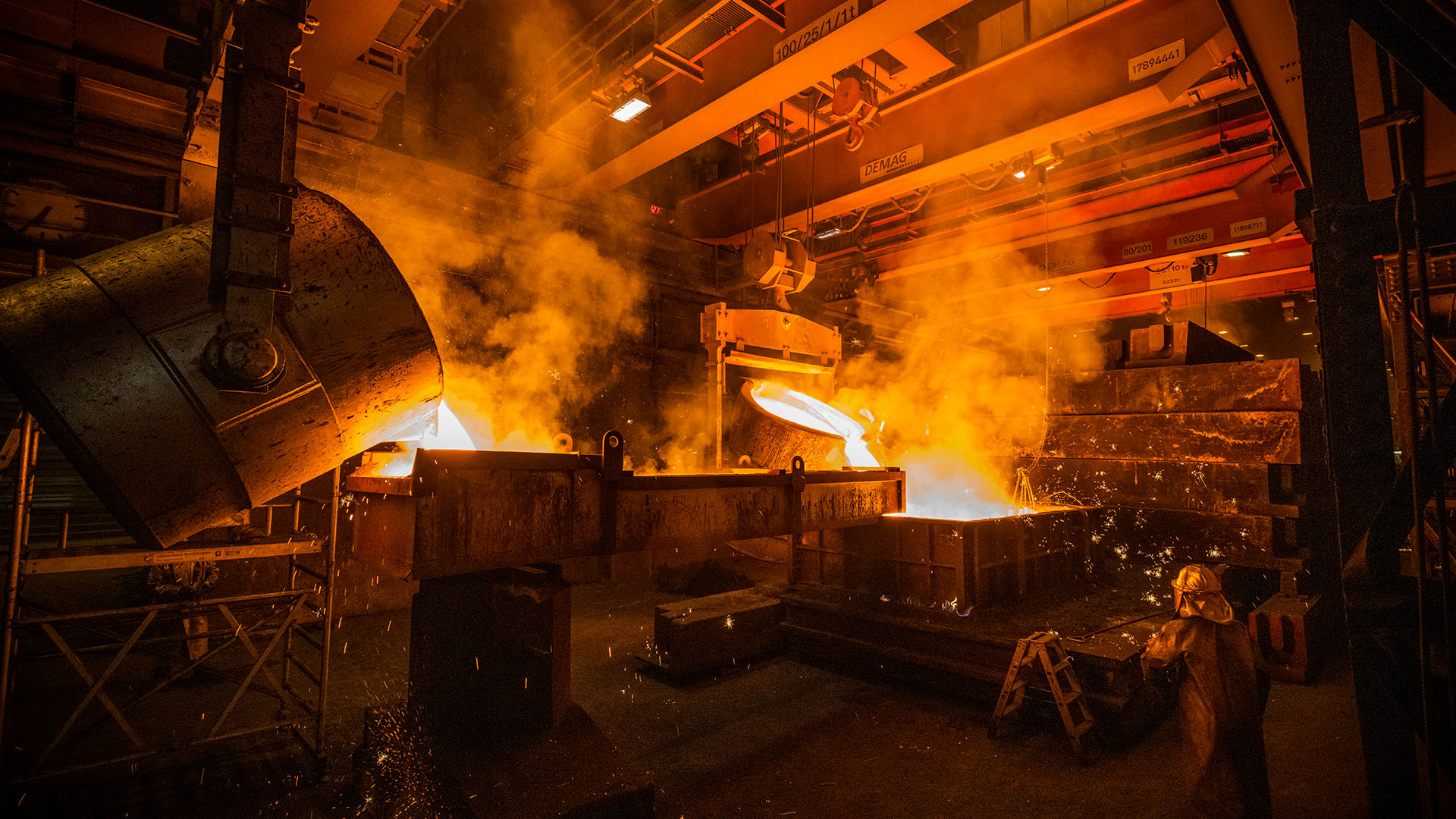The image depicts a fiery industrial forge scene inside a factory. Central to the image are two substantial metal cauldrons, with the one on the left angled slightly to the right as it pours molten, fiery liquid into a container below. Just behind it and to the right, another cauldron also tilts forward, pouring its molten contents into the same receptacle. The bright, orange molten liquid, almost resembling lava, emits luminous white and orange hues, with smoke billowing dramatically from the pouring sites. A metal pipe-like structure connects the two cauldrons, enhancing the mechanical complexity of the scene. Adjacent to the container, there's a small step ladder, beside which stands a person donned in a protective suit and helmet, overseeing the operation. Above, a network of metal bars and wires crisscross the ceiling, from which various machinery parts dangle, while red beams and additional metal structures frame the room, adding to the industrial atmosphere.